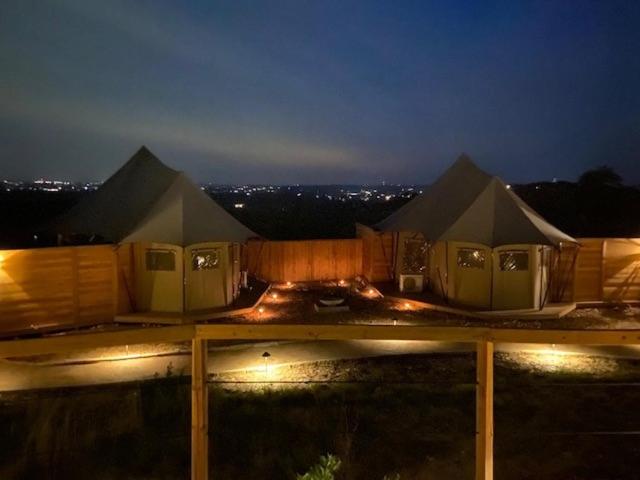The image captures a night scene at a temporary campsite, framed by a light wooden fence that features two symmetrical structures at its center. These structures, designed with olive green, tent-like canvas roofs and tan doors, each flanked by two small plastic windows, evoke a provisional setup. A dark stone pathway, adorned with small solar lights, runs in front of the structures, guiding the way through the campsite. Between the structures lies a dirt area illuminated by several candles, adding a warm glow to the scene. The fence extends horizontally across the image, defining the boundaries of the campgrounds. Behind the tents, beyond an orangey-wood fence that runs from left to right, there's a backdrop of dark silhouettes, possibly trees, under a deep purple and blue night sky. In the distance, twinkling city lights dot the horizon, contrasting with the encroaching darkness around the campsite. The image appears to be taken from just behind another light wooden banister or platform, indicated by its delicate structure with black strings and surrounding foliage.